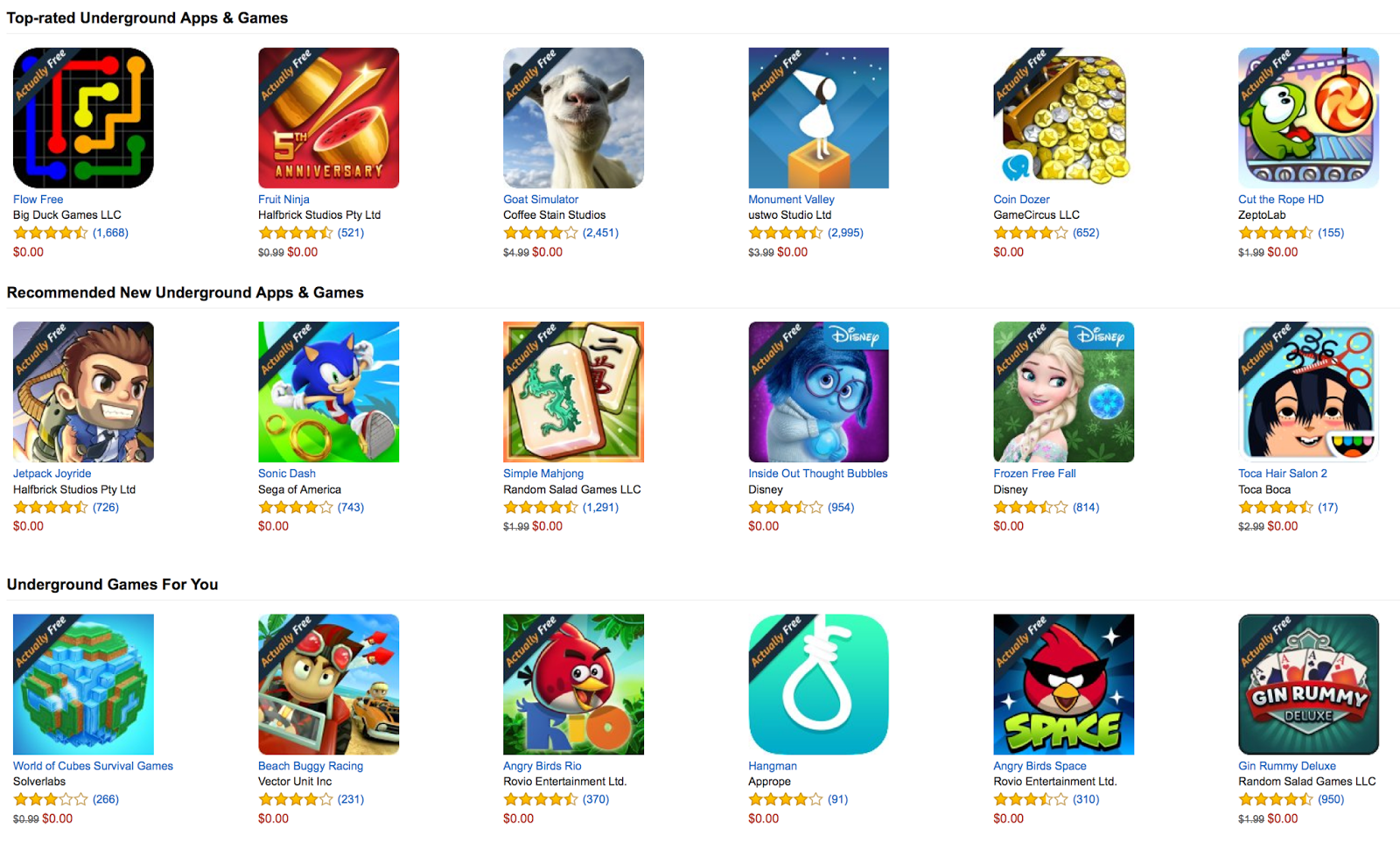Here is a refined and detailed caption for the image:

"A screenshot from a game application website showcasing a selection of 18 vibrant and colorful mobile games. Each game is represented by an illustrative icon and is accompanied by its title, the developer company name, a star rating, and the number of contributing reviewers. Additionally, the price of each game is displayed beneath its respective information. These titles are designed for mobile platforms, including smartphones and tablets."